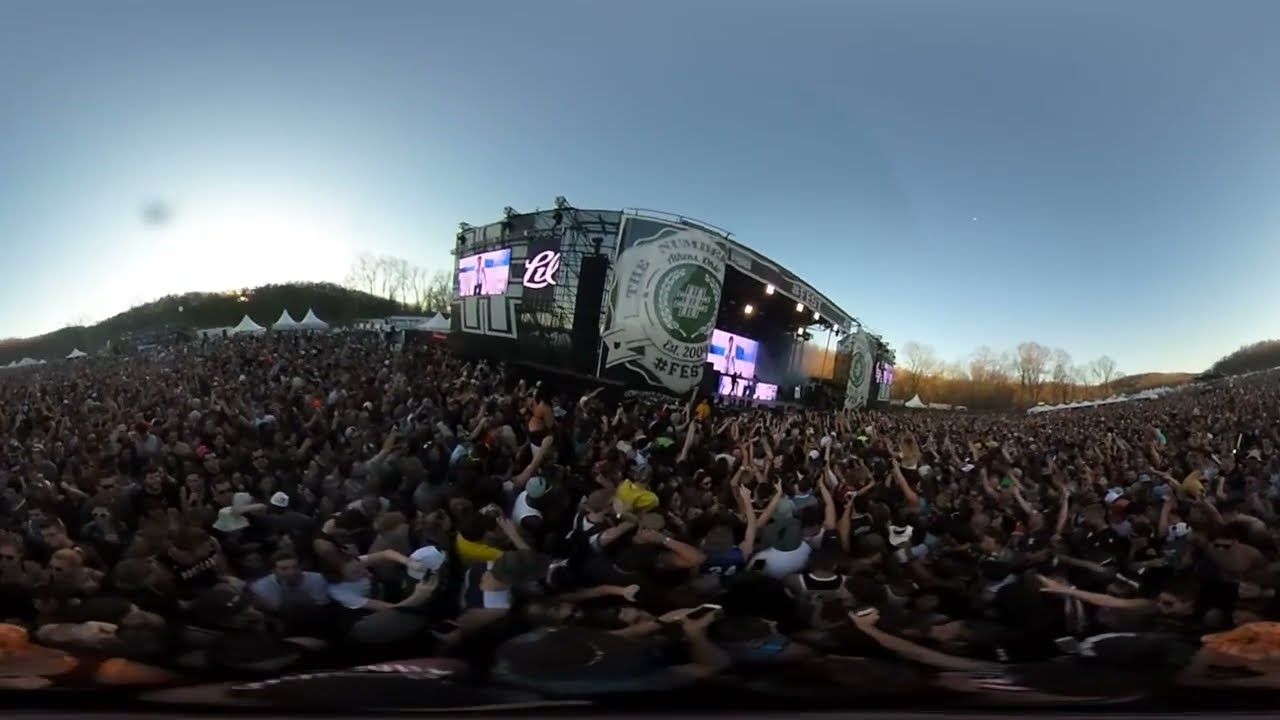The photograph captures a vibrant, panoramic view of a music festival in a sprawling outdoor venue. In the foreground, a massive crowd stretches across the entire width of the image, their raised arms and enthusiastic expressions conveying their excitement. The stage, positioned centrally but slightly angled from the left side of the audience, is equipped with large screens displaying a performer in a white shirt and dark pants against a beach backdrop. Overhead, the dull blue sky is tinged with white from clouds and sunlight.

A notable feature is the large badge on the left side of the stage, bearing a green circle framed by two long, narrow, grain-like plants, with the text "Est 2004, #Fest" in white. Rolling hills lush with trees form the background, enhancing the natural beauty of the setting. Scattered tents and canopies, predominantly white, are visible in the distance, adding to the festival atmosphere. The stage itself has a gray floor and a black ceiling, with lights illuminating the performer. The various elements combined—boisterous crowd, detailed stage, scenic background, and clear sky—create a dynamic and detailed depiction of the lively event.